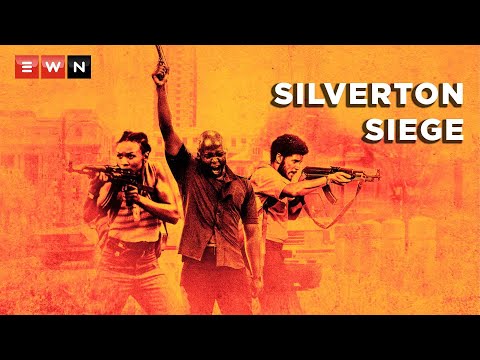The poster appears to be an advertisement for an action movie titled "Silverton Siege." It features three central figures, all prominently armed and emanating a sense of urgency and aggression. The background predominantly showcases muted hues of orange, red, and yellow, with a faint cityscape visible behind the characters. 

At the top left corner, the letters "EWN" are displayed, with the "E" and "W" appearing in white on red squares and the "N" in white on a black square. The film's title, "Silverton Siege," is boldly printed in white letters with a black shadow on the top right corner of the poster. 

The central figure is an angry black man holding a pistol high in the air, his mouth open as if shouting. Flanking him on either side are two other figures: to his left, a bearded black man dressed in a t-shirt and armed with an automatic weapon, and to his right, a woman with her hair pinned up, also dressed in a striped t-shirt and wielding a similar automatic rifle. The entire image is framed by black borders at the top and bottom. The overall composition is dynamic, echoing themes of intensity and conflict typical of an action movie.